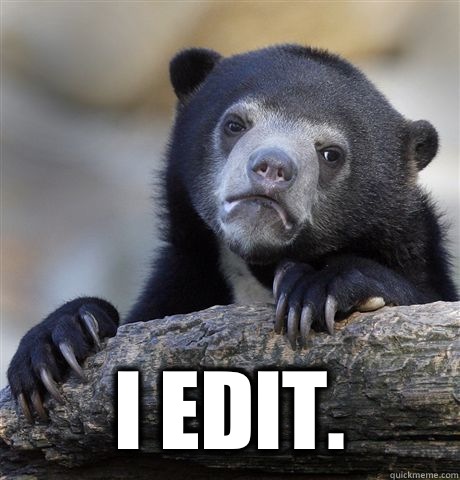This meme features a melancholy-looking animal, possibly a bear, with predominantly gray fur. The area around its eyes is lighter, contrasting with its grayish nose. Its mouth is downturned, enhancing its sorrowful expression. The animal grips a log with its long claws, filling the lower third of the image. The background is blurred out, keeping the focus on the animal. Overlaid in white, capital letters, the caption reads, "I EDIT."